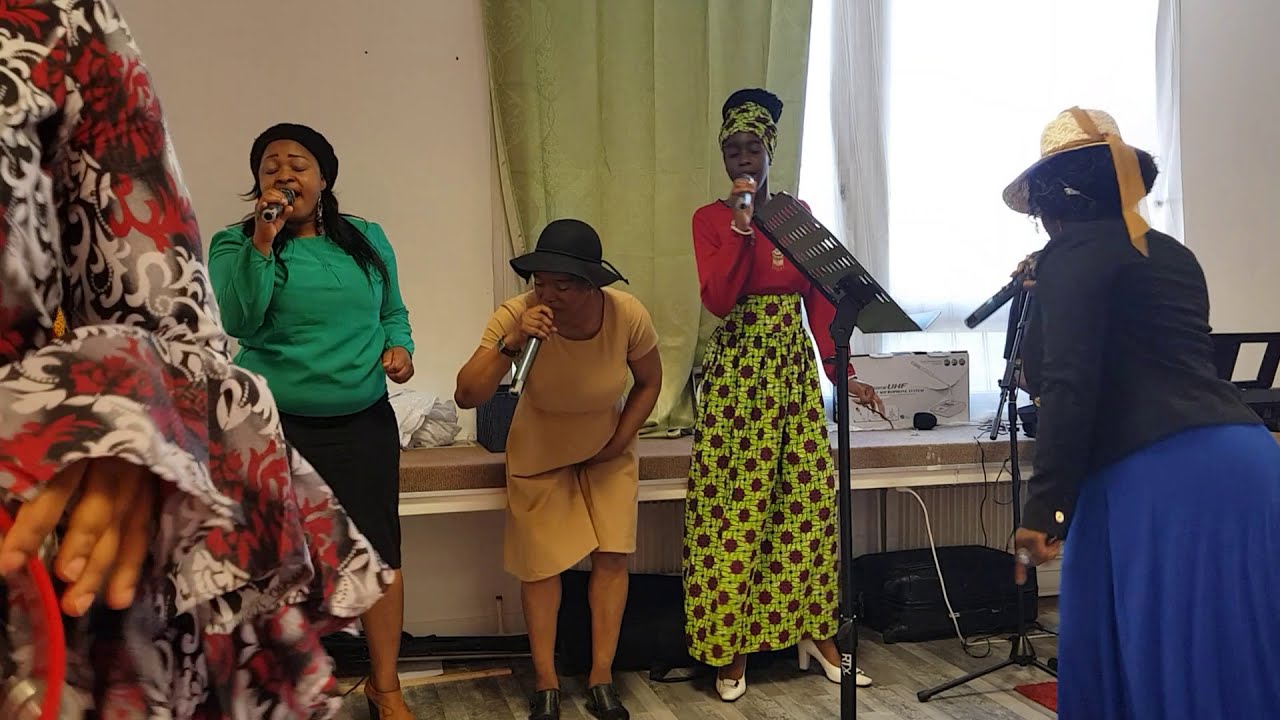In this photograph, four African American women are captured in the midst of singing, each holding a microphone in their right hand. On the far left, only an arm adorned in an elaborate garment with rich fabric can be seen, hinting at another individual partially outside the frame. Moving inward, the first visible woman wears a green shirt paired with black pants or a skirt and is actively singing into her microphone. Next to her, a woman with a yellow-orange shirt and a black hat is slightly crouched over, seemingly clutching her stomach as she sings. The third woman, standing taller and younger in appearance, is dressed in a red shirt and a high-waisted green skirt with brown patterns, complemented by a green headband that matches her outfit. To the far right, the fourth woman has her back to the camera, sporting a black shirt, blue skirt, and a hat. She appears to be leaning slightly forward while singing. Behind this group, the setting includes a table with computer equipment and possibly some luggage underneath. There is also a large window suggesting daylight outside, flanked by green drapes. The backdrop and detailed attire contribute to a vivid and dynamic scene of communal singing.